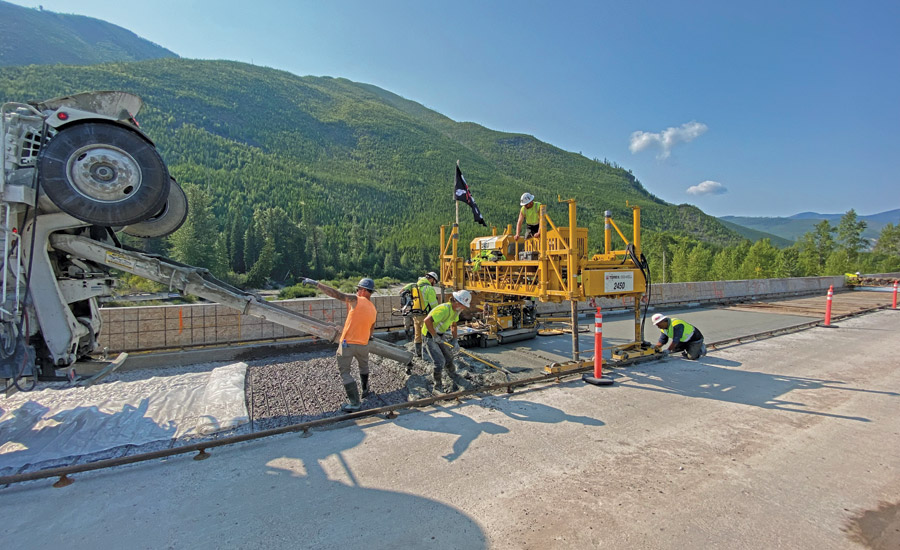The photograph captures a bustling scene of a road construction crew actively working on a highway surrounded by verdant green mountains and a clear blue sky dotted with a couple of clouds. Centered on the left side of the image, a concrete truck is pouring cement, directed by a construction worker in a bright orange sleeveless shirt, blue hard hat, khaki pants, and black mud boots. Adjacent to him, another worker dressed in a neon green construction vest and white hard hat smooths the freshly poured concrete with a rake, wearing black pants and wet boots. Towering over the scene on the right is a yellow scaffolding with another worker on top in similar neon green attire and white hard hat, supervising the work below. A blue, red, and white flag flutters near him. On the ground below the scaffolding, a worker sits meticulously refining the smoothed cement, hinting at recently completed work further down the road. Scattered orange cones mark the work area, while the lush backdrop of hills adorned with leafy trees enhances the vibrant, orderly chaos of the construction site.